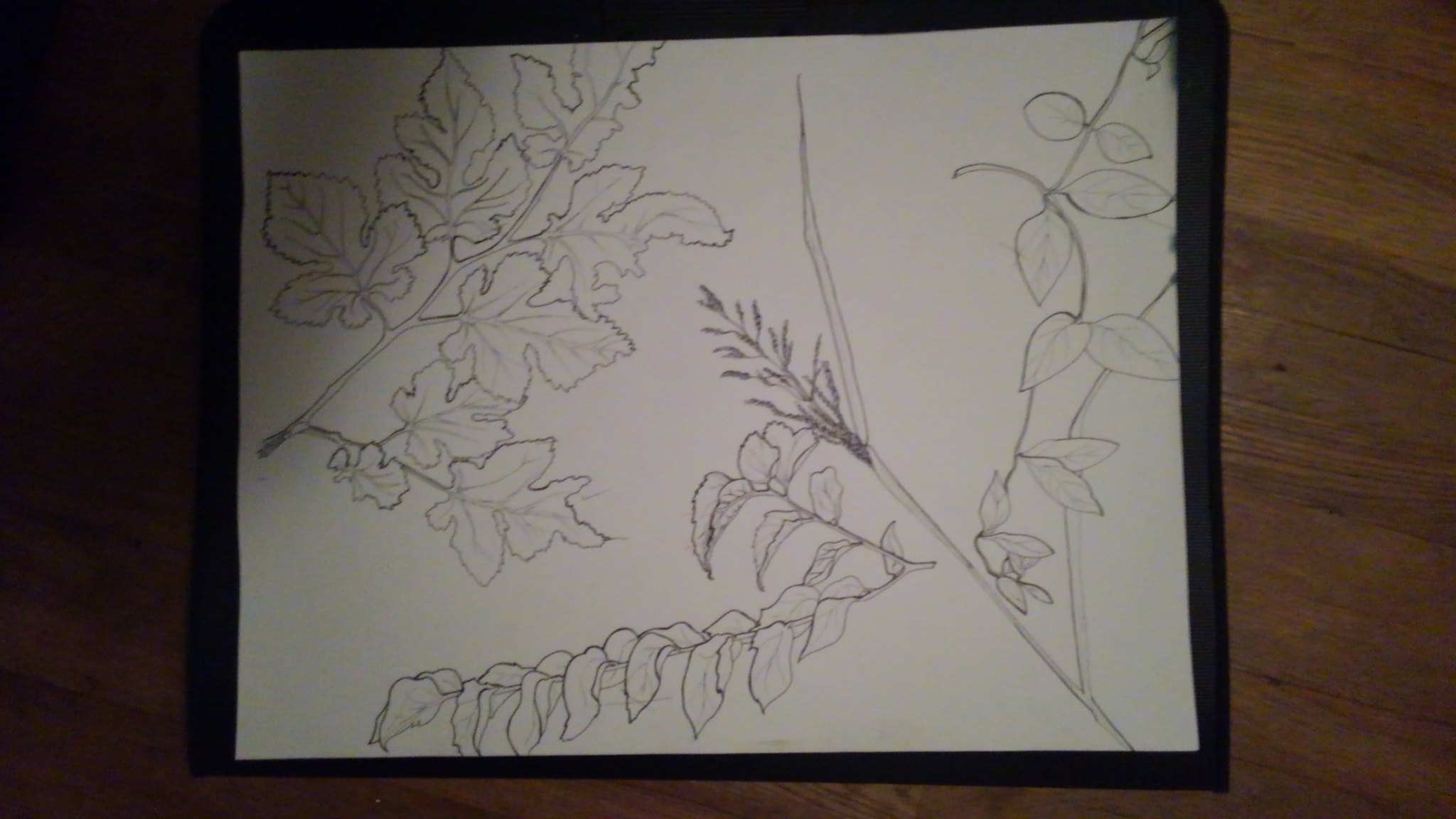The image showcases a detailed drawing of various types of leaves attached to stems, made on white paper. The paper is placed against a black background, which in turn rests on a dark brown wooden surface. In the upper left corner of the drawing, there are eight oak leaves attached to two main stems. At the center of the composition, there are smaller leaves that resemble miniature elephant ear leaves. Just to the right of these leaves, there is a stalk that looks like wheat. Above this wheat-like stalk, about a dozen normally-shaped leaves are intricately illustrated, adding to the diversity of the foliage depicted in the drawing.